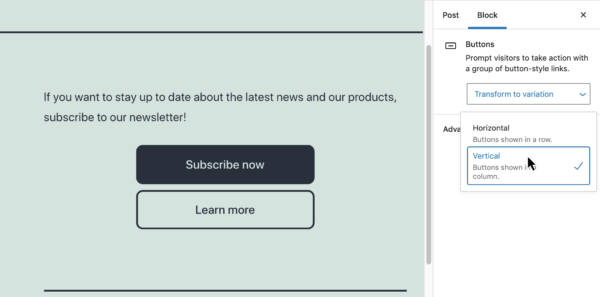In the image, we see a screenshot of a subscription prompt. A light green rectangular box prominently features the text: "If you want to stay up to date about the latest news and our products, subscribe to our newsletter." Above this text is a thin, dark green horizontal line adding subtle separation. Below the message are two action buttons: one black button with the white text "Subscribe Now," and beneath it, a light green button labeled "Learn More." Further down, another dark green horizontal line is present.

To the right, there is a small white box in the top left corner of a white page. This box contains the bold black text "Post," and below it, there is an underlined blue link labeled "Block." Beneath these links are various buttons prompting visitors to interact. A button with a pull-down option reads "Transform to Variation," followed by a second button within a box. Horizontal buttons are displayed in a row beneath this, within a rectangular box highlighted in blue. Below it, black text reads "Buttons Shown Column," accompanied by a blue checkmark.